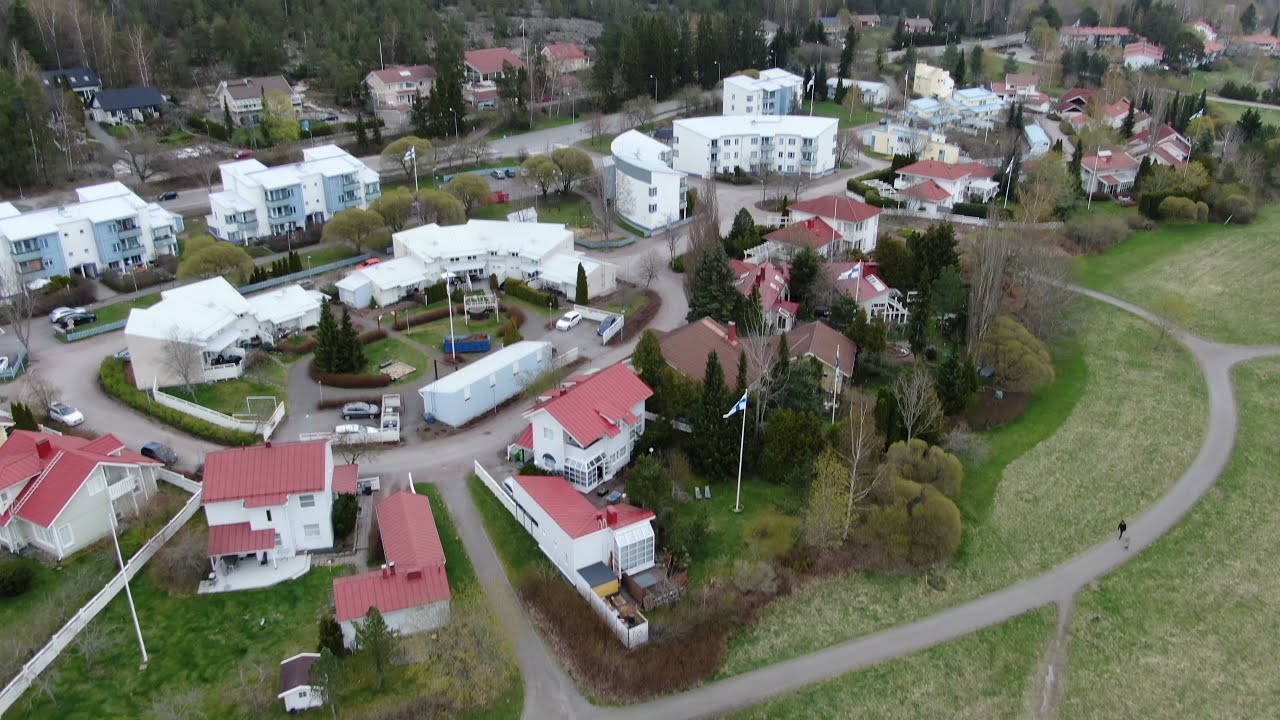This aerial photograph captures a detailed and vibrant view of a residential neighborhood. The majority of the dwellings are white homes with distinct red roofs, varying from one to two stories. Larger white and blue three-story buildings, which appear to be apartment complexes, are scattered around, adding to the urban density. The neighborhood is crisscrossed with gray streets and pathways, featuring a prominent circular road in the center surrounded by both houses and apartments. In the bottom right, a curved walkway adorned with green fields and trees showcases a serene part of the community. Trees, both lush and bare, line the roads and enhance the verdant landscape, which is interspersed with patches of grass in the yards. The image also reveals people engaging with the space: a man can be seen walking along a path at the bottom right, as well as potentially a person with a dog on another path. Vehicles of various colors, including red, white, black, and blue, populate the streets and parking areas. The entire scene is set against a backdrop of cream and terracotta buildings, complemented by commercial-looking structures sprinkled throughout, affirming the area as a predominantly residential neighborhood with pockets of mixed use.